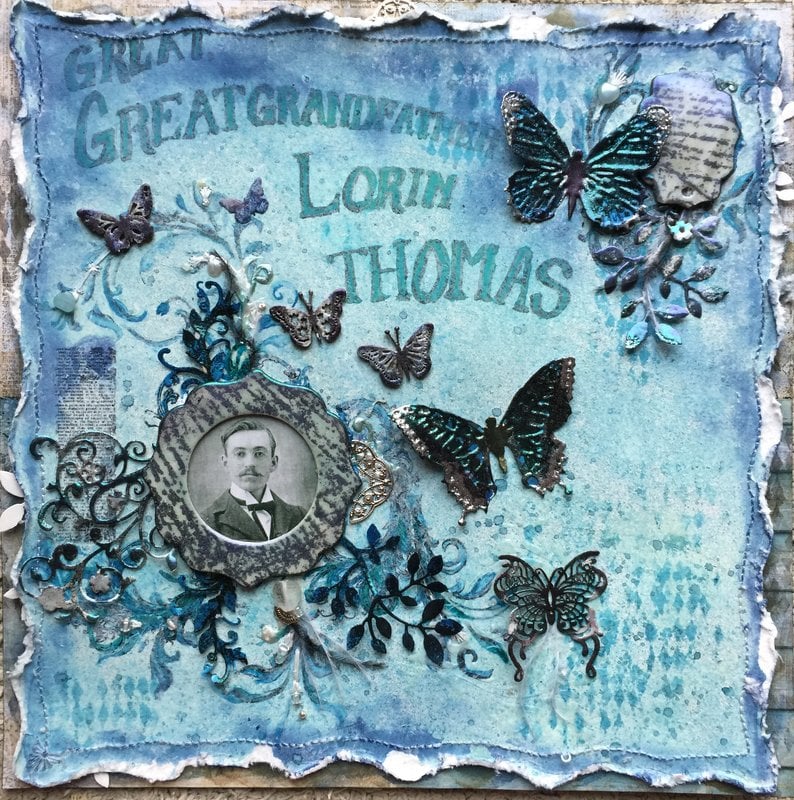This image depicts a weathered, possibly 19th-century, fabric mural or framed portrait mounted on a wooden surface. The mural features a prominently blue background in various shades, including hints of violet, and showcases seven butterflies of varying sizes, along with twining vine-like and floral patterns. In the upper left corner, the text "Great Great Grandfather Lauren Thomas" is printed in a different shade of blue. In the lower left corner, there is a black-and-white photograph of a mustachioed gentleman with glasses, wearing a white collared shirt with a black tie and a suit. The photo is encased in a circular frame that resembles a flower with vines, adding to the vintage aesthetic. The overall scene gives a strong impression of being a commemorative piece, reflecting the historical era with both the style and the condition of the materials used.